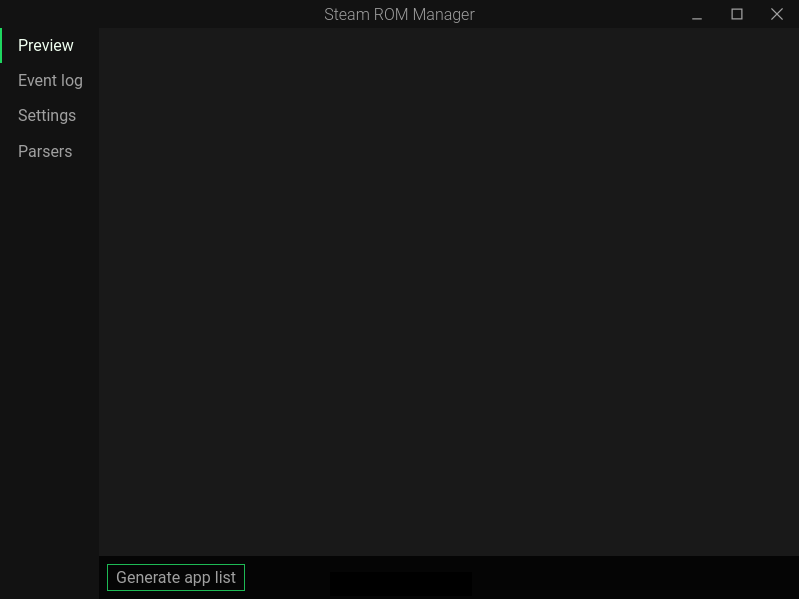The image showcases a software interface for "Steam ROM Manager." The left side features a solid black background with the word "Preview" in white at the top, followed by "Event Log Settings and Parsers" in similar white text. Central at the top, "Steam ROM Manager" is displayed in light gray text. The top right corner includes a series of standard window controls: a minus sign, an outlined box, and an 'X,' all in gray. The interface's background blends from a dark brown in the middle section to black on the left and bottom edges. At the bottom center, there's a neon green outlined box with "Generate App List" written in gray text. The overall color scheme contrasts light gray text against dark backgrounds, with the "Preview" section distinctly in white for emphasis.